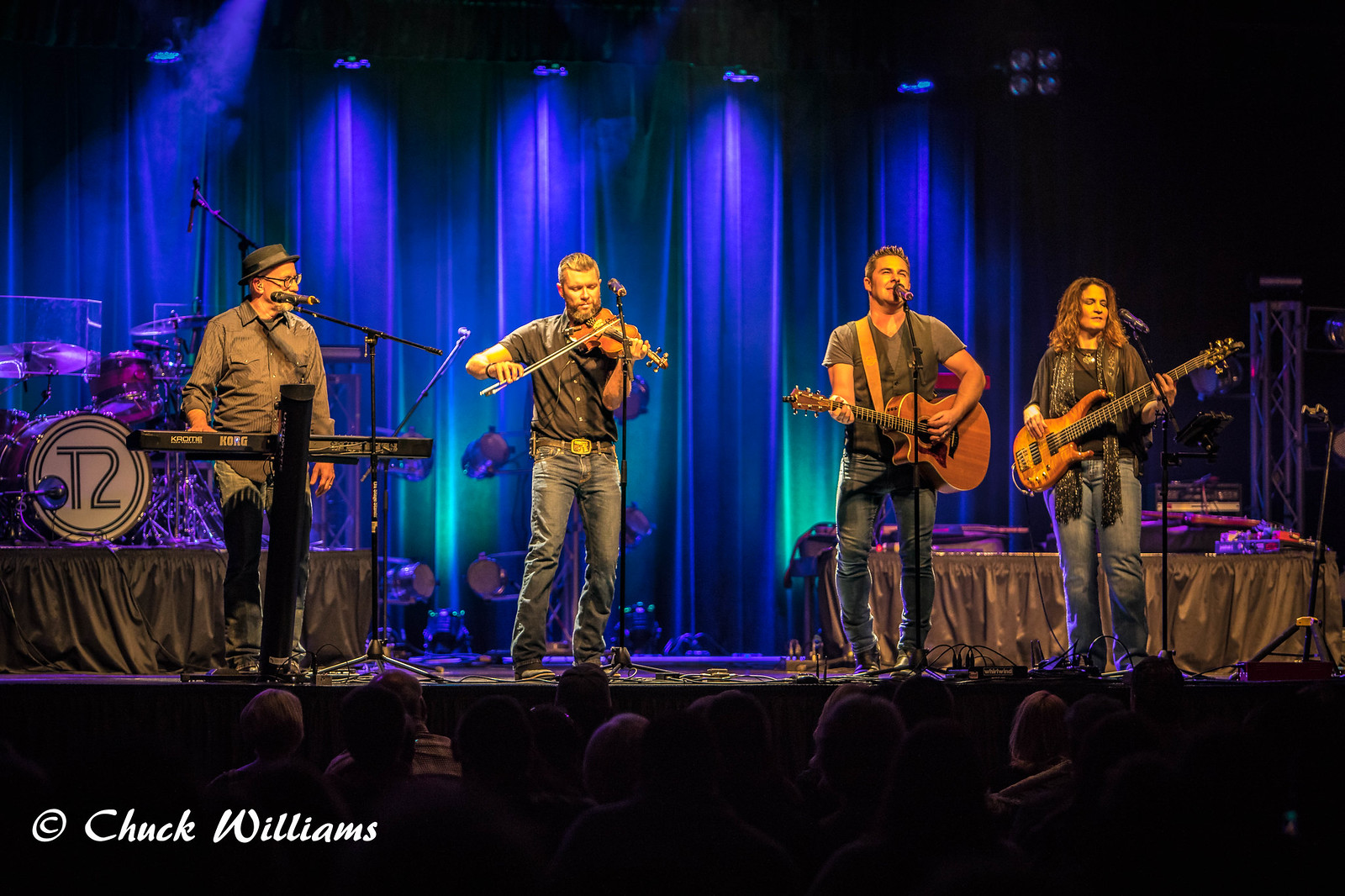This photograph captures a vibrant live performance of a musical group on a dimly lit indoor stage, bathed in blue lighting from behind. The stage backdrop features blue drapes, and various dark tones dominate the scene, including black, gray, and brown, complementing the instruments and attire. There are four performers on stage:

- To the far left, a man wearing a black cap, gray shirt, and black jeans is playing a keyboard, standing in front of a drum set encased in a plexiglass barrier.
- Next to him, another man in a black shirt and blue jeans is playing a violin.
- The third performer, also a man, dressed in a gray shirt and blue jeans, is singing into a microphone while holding an acoustic guitar with a shoulder strap.
- On the far right stands a woman wearing a black jacket and a gray scarf, playing a brown electric bass guitar.

Spectators’ heads are faintly visible in the shadowed audience area, all facing the stage. An inscription that reads "Chuck Williams" is located at the bottom left of the image.